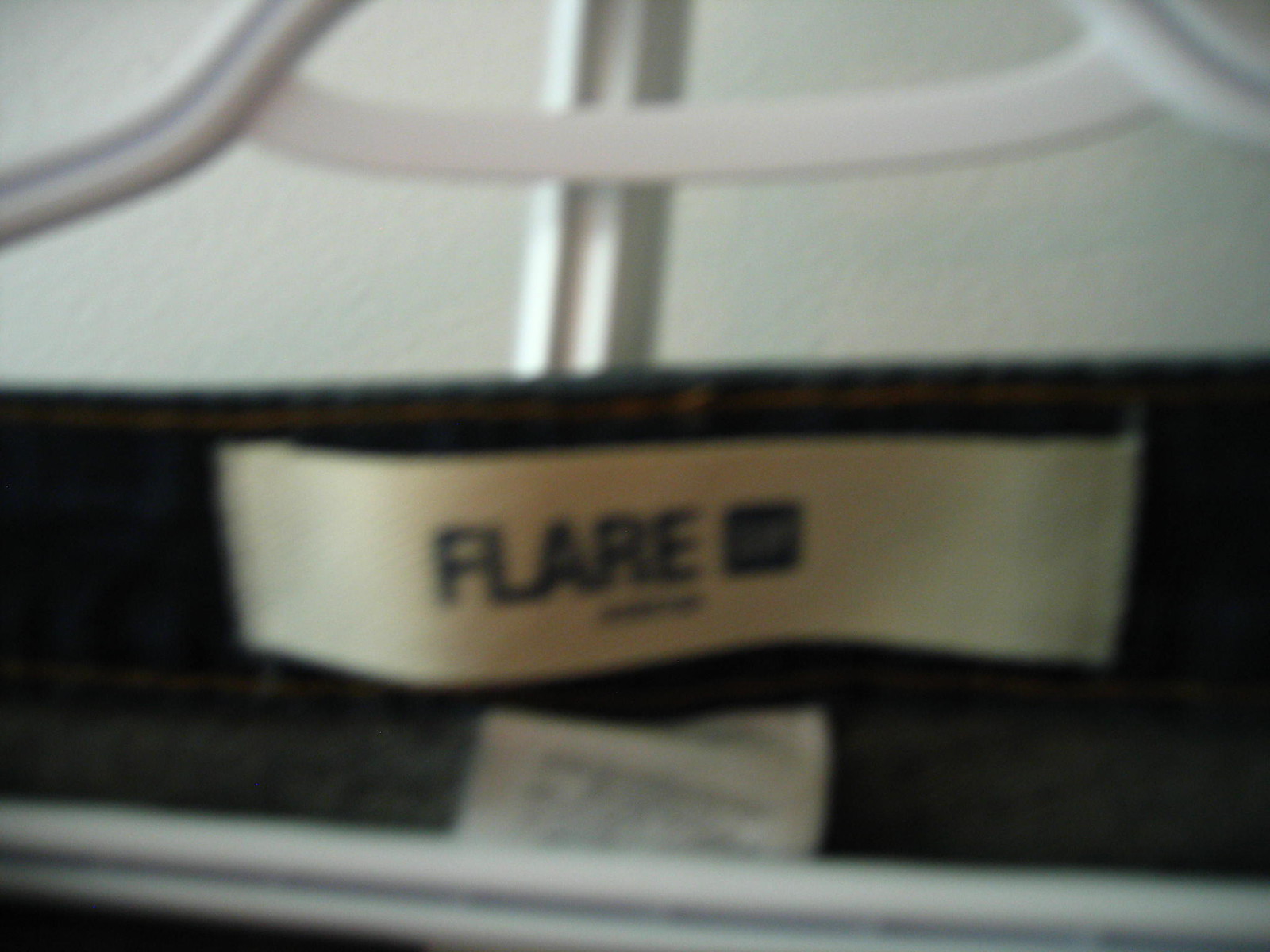The image is a blurry, low-resolution color photograph with poor lighting, making it challenging to distinguish the details clearly. The focal point of the image is a close-up of the neck area of a dark-colored piece of clothing, which is either very dark brown or black. This garment is hanging on a white plastic hanger, which is partially visible with two curved top edges that converge beyond the upper boundary of the photo and a horizontal bar at the bottom.

In the center of the image, there's a slightly curved, rectangular fabric tag that is off-white or whitish in color. Prominently displayed in capital letters is the word "FLARE" written in black. Beside this, there is a small, dark blue or black square containing some unreadable fake writing, likely intended as a logo. Beneath the word "FLARE," there is additional small black lettering that is also indiscernible due to the blur. Another tag is visible below the main label; it is more square-shaped and has very thin writing, which, again, is not legible.

The stitching on the clothing is a golden or brownish color, hinting at detailed craftsmanship. The backdrop consists of a grey background and another brightly colored bar emerging from behind the garment, adding more depth to the image. The interior fabric of the clothing appears slightly lighter, giving a grayish impression with white splotches.